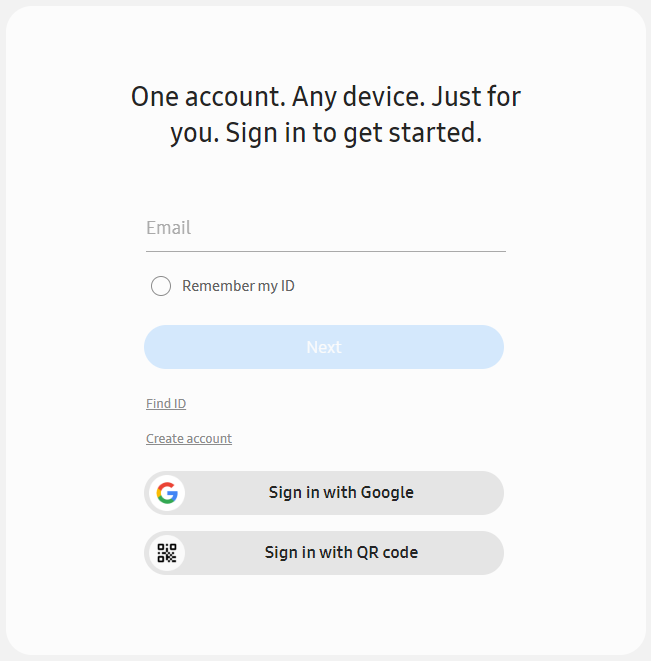The image depicts a sign-up page with a light gray background. At the top center of the image, bold black text reads: "One account and a device just for you. Sign in to get started." Below this heading, there is a text field labeled "Email." Adjacent to this is a checkbox labeled "Remember my ID." Below the email input section, there is a blue "Next" button with white text; however, this button appears slightly transparent because no email has been entered yet.

Underneath the "Next" button, on the left side, are two gray, underlined links: "Find ID" and "Create Account." Further below, there are two sign-in options. The first button reads "Sign in with Google," featuring a black text on a gray background. To the left of this text is a white circular icon with a colorful 'G' consisting of red, yellow, green, and blue segments.

The second button at the bottom reads "Sign in with QR Code," designed similarly—with black text on a gray background. On the left of this text is an icon of a QR code, rendered in black against a white background.